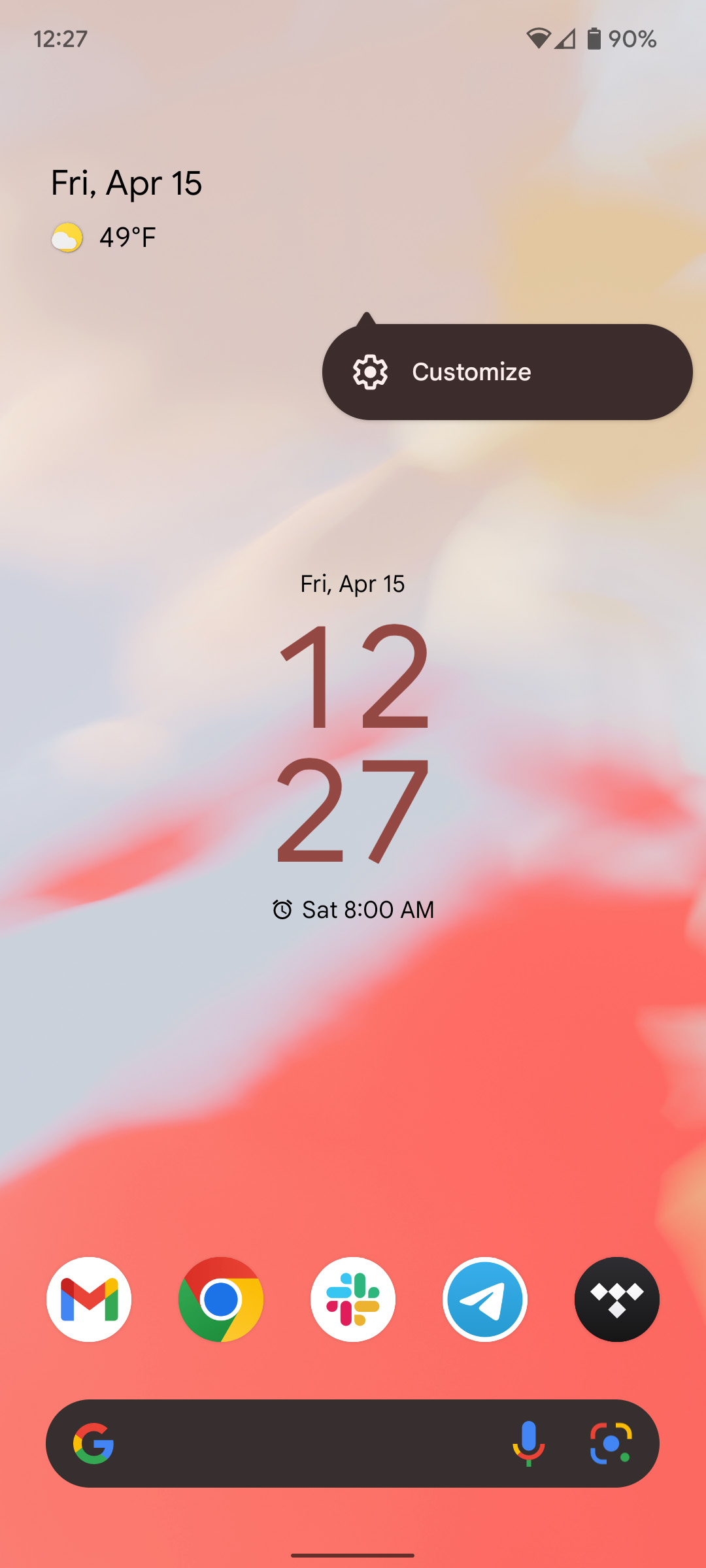This is a detailed screenshot of a phone home screen, featuring a vibrant background with a gradient cloud effect. The gradient starts with a pinkish peach hue at the top, transitions into shades of blue, yellow, and white, and then shifts back to pink toward the bottom. In the top left corner, the time is displayed as 12:27 PM, while the top right corner shows the Wi-Fi signal strength, cellular network bars, and a battery icon indicating that 90% battery life remains. The current date, "Friday, April 15th," along with the weather condition "partly cloudy" and the temperature "49°F," is also noted in the top left corner.

Below this, an oval-shaped rectangle, approximately an inch long and a quarter-inch deep, appears on the screen. This oval rectangle, featuring a brown color, houses a settings symbol and the word "Customize."

Dominating the middle of the screen is a larger, clear display of the date "Friday, April 15th" and the time "12:27 PM." Directly below the time, there's an icon of an alarm clock indicating a scheduled alarm set for Saturday at 8 AM.

The bottom of the screen hosts a row of app icons, including Gmail, Chrome, a multicolored flower-like icon, a blue circle with a white arrow, and a brown circle with four dots. Beneath these icons lies the Google search bar, offering quick access to internet searches.